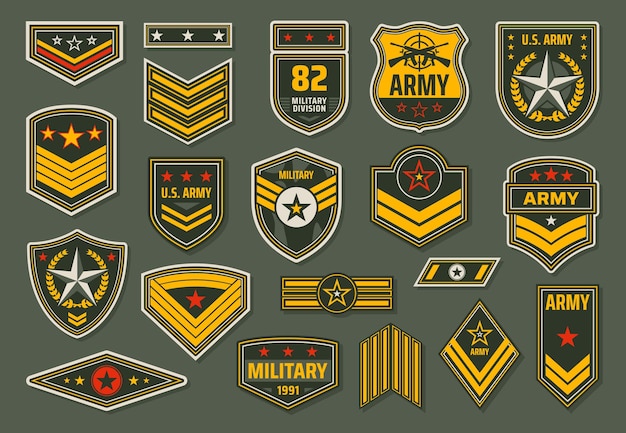This image showcases a detailed artist's rendering of various U.S. Army and military badges on an olive green background, consistent with a vector design for Armed Forces Day. The badges are spread across multiple rows, with five badges per row, each representing different military ranks and divisions. Key details include a prominent pentagon-shaped badge resembling a baseball home plate in green, yellow, and red located in the upper left-hand corner. In the center, a badge with the number '82' in yellow, accompanied by 'Military Division' in white, stands out. Several badges feature inscriptions such as "U.S. Army," "Military 1991," and "82nd Military Division." The badges, varying in shapes and sizes, incorporate colors like gold, red, dark forest green, and occasional spots of gray. Symbols include stars, shields, stripes, and crossed rifles, providing a comprehensive visual array of military insignia.